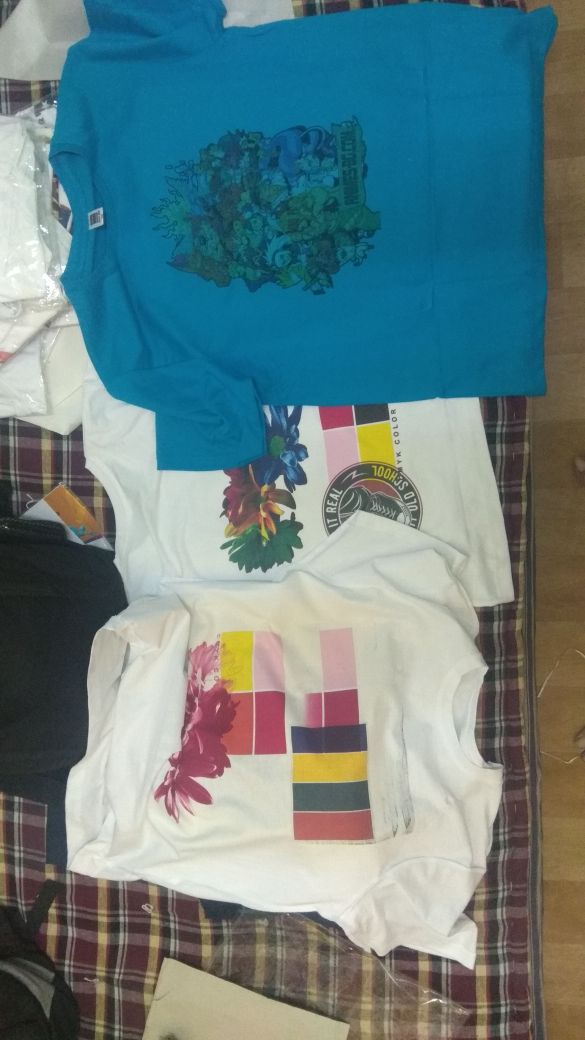This photograph, taken from a high angle, captures a wooden floor with a red and yellow plaid blanket draped over it. On top of the blanket, various articles of clothing are scattered, predominantly featuring t-shirts. In the upper portion of the image, a blue t-shirt with an intricate and busy design—possibly cartoon characters or small figures—is prominently displayed. Below it, overlapping slightly, are two white t-shirts. One features a series of squares in vibrant hues of purple, pink, orange, yellow, and black, with dark and light pink flowers situated at the bottom when properly oriented. The other white t-shirt showcases an array of multicolored flowers—green, brown, blue, orange—and rectangular, color-block designs. Additionally, other white articles of clothing peek out from under the more visible shirts, though their details remain obscure. Some random papers and indistinct clothing items also fringe the edges of the photo.